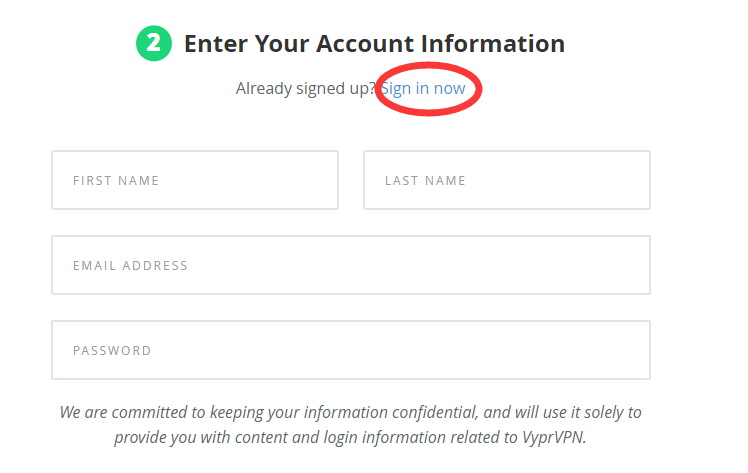This is a detailed depiction of a sign-in/sign-up page for VyprVPN, based on a voice-captioned image. 

The page features a prominent "2" enclosed within a green circle, indicating the step number, with adjacent black text instructing users to "Enter your account information." Below this instruction, a message for existing users reads "Already signed up? Sign in now," with "Sign in now" highlighted in blue text and encircled by a red oval for emphasis.

The form includes several entry fields. At the top, two side-by-side fields, each surrounded by gray borders, request "First Name" in the left field and "Last Name" in the right. Directly beneath these fields are additional inputs labeled "Email Address" and "Password." At the bottom of the form is a disclaimer in italicized font that assures users, "We're committed to keeping your information confidential and will use it solely to provide you with content and log information related to VyprVPN."

The rest of the screen is primarily white, though it's unclear whether the image is a photograph of a phone screen or a screenshot viewed on a computer. The ambiguity suggests it may be a pop-up screen on a computer.

![Sign-In/Sign-Up Page for VyprVPN](URL to JPEG if available)